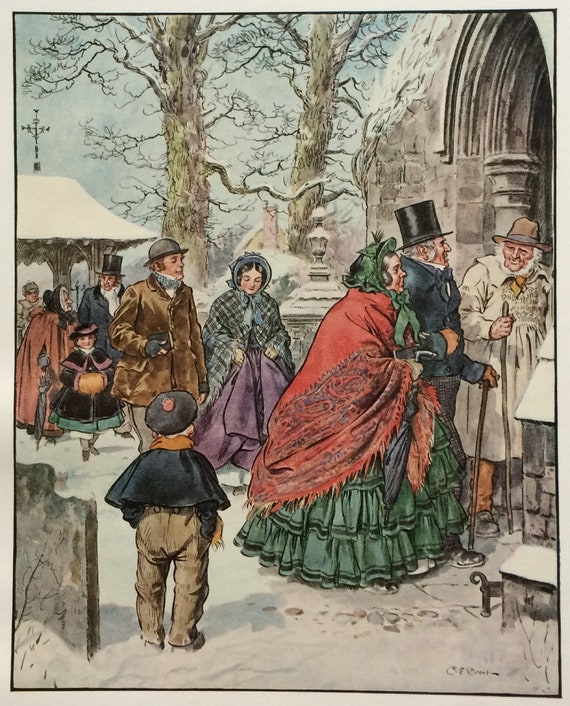This artwork, a painting or intricate sketch signed in the bottom right-hand corner by an artist named C.E.D. Brock, depicts a bustling winter scene in a quaint, snow-covered town. Central to the image is an ornate stone church with a grand, columned archway. A crowd, dressed in Victorian-era attire, is filing into the church. Leading the group is an elderly man with a cane, followed by an older couple; the man donning a black top hat while the woman wears a wide green dress, a red shawl, and a green bonnet. Nearby, a little boy in a black shawl and hat stands next to a tombstone, observing the scene. Other townsfolk, including a younger couple, a little girl in a blue and pink dress, a woman in a blue jacket, and several men in winter coats and top hats, add to the lively scene. The background features two large, snow-dusted trees, a yellow house with a red brick chimney, and possibly a fountain, all contributing to the serene, frosty atmosphere of a bygone winter day.